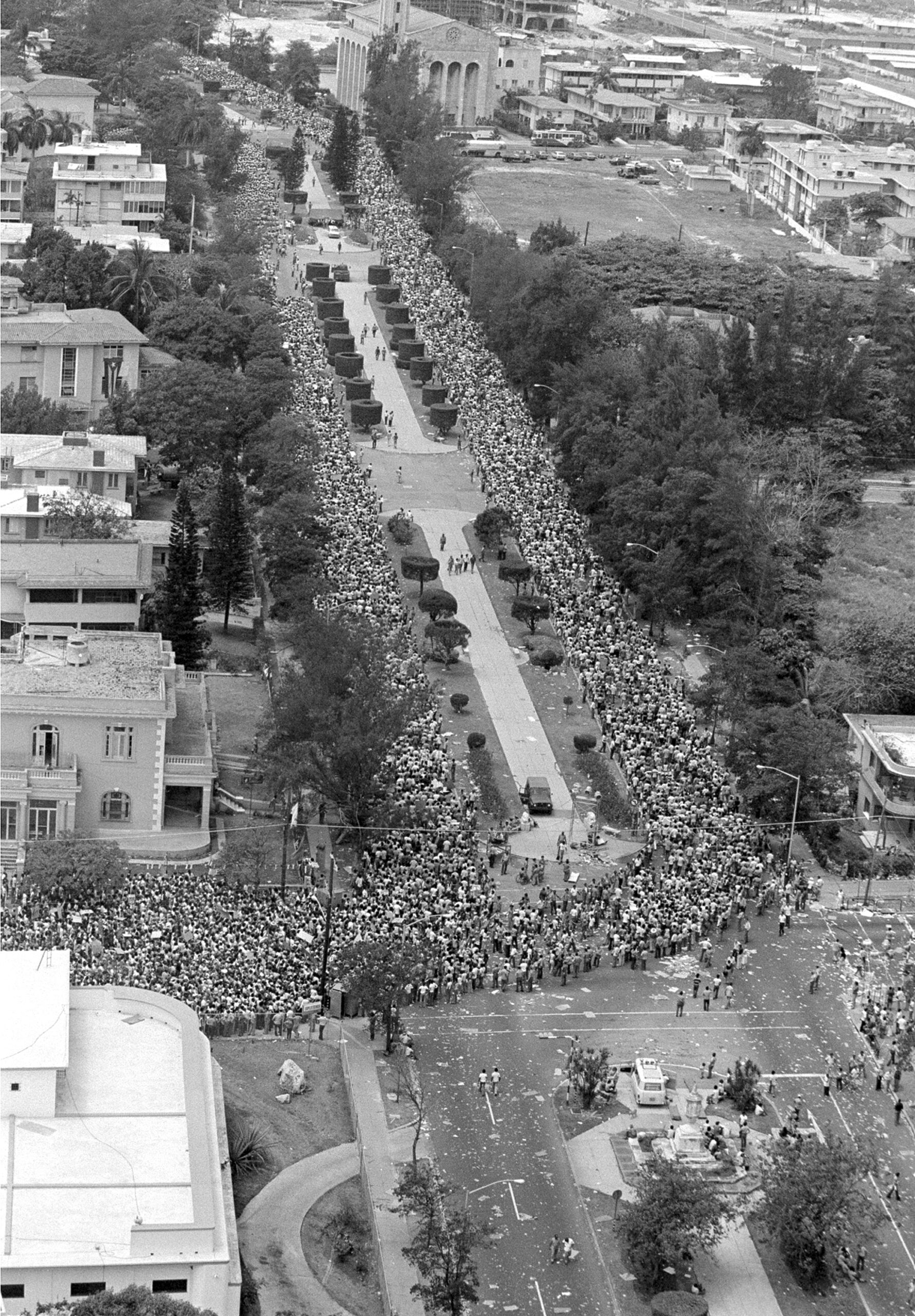This black and white aerial photograph captures a historic moment, likely the "I Have a Dream" speech by Martin Luther King Jr. at the Lincoln Memorial in Washington, D.C. The image showcases a massive crowd, possibly numbering tens of thousands, gathered in the National Mall area. The crowd is organized into two continuous streams marching down parallel roads, separated by rows of manicured shrubs and flanked by tall trees on both sides.

In the distance, a large, columned building, presumably the Lincoln Memorial, stands out prominently, surrounded by mid-20th century buildings that might be residential or business in nature. The streams of people converge from all directions, creating an impressive procession that flows from the center of the image down to the left and right edges of the frame.

The participants' white shirts stand out, and scattered among them are various signs. There is a noticeable police presence, particularly in the bottom left and right corners, maintaining order around the perimeter. In the lower right corner, a small group of individuals appears to be managing a mess on the street, while others look on. Overall, the scene is peaceful, highlighting the significant turnout and the orderly nature of this historic gathering.